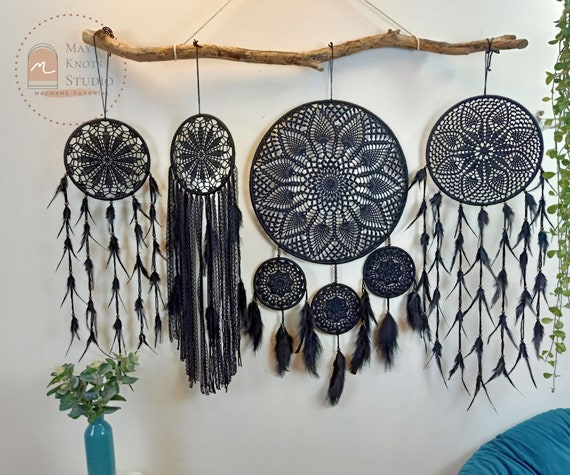The photograph features four intricately woven Native American dreamcatchers, each crafted with black lace and adorned with various feathers and other decorative elements hanging down towards the bottom. These dreamcatchers are suspended from a piece of driftwood, which is itself secured to a white wall via a white string. In the top left corner, a prominent watermark reads "Mae Knott's Studio," featuring a stylized white "M" set against a coral arched background. In the bottom left corner of the image, a turquoise vase filled with eucalyptus leaves adds a touch of natural greenery. On the right side, a green hanging plant can be partially seen, adding more natural elements to the composition. The bottom right corner showcases a glimpse of a turquoise chair, partially obscured, contributing to the overall setting's cohesive color scheme and tranquil atmosphere.